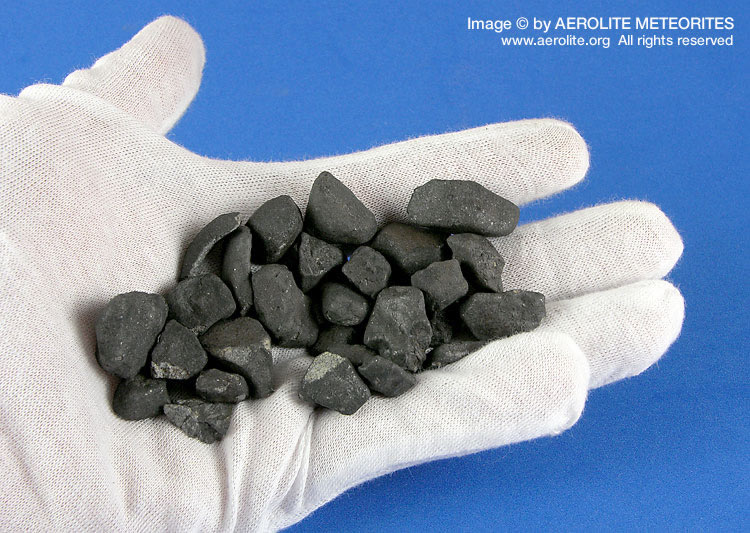The image depicts a left hand wearing a white cotton glove, holding a cluster of small, dark gray or black rocks, possibly meteorites. The hand is extended and open, with all fingers visible, set against a vivid blue background. The copyright notice is displayed prominently in the top right corner in white text, reading "IMAGE © AEROLITE MEDIA RIGHTS" with "www.aerolite.org" and "All Rights Reserved" underneath in a smaller font. The arrangement draws attention to the contrast between the white glove, the dark rocks, and the blue backdrop.